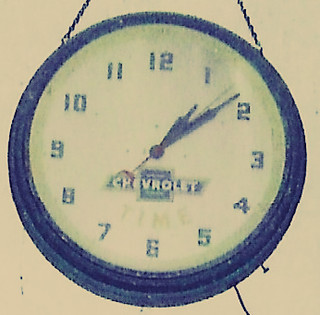A vintage Chevrolet wall clock with an aged and faded appearance is the focal point of the image. The clock features a classic design with a white face and bold, black numbers ranging from 1 to 12. It has black hour and minute hands, along with a slim black seconds hand. A distinctive Chevrolet logo in white font is prominently displayed on a small black square towards the center of the clock, with the word "Time" written just below it.

The clock is encased in a black body, giving it a sturdy frame. Unique to its design are the chains attached to the left and right sides at the top, serving as the hanging mechanism. Additionally, small stakes protrude from the bottom-right side of the clock, adding to its rustic charm. The background features a beige color, enhancing the vintage, slightly worn-out feel of the overall scene.